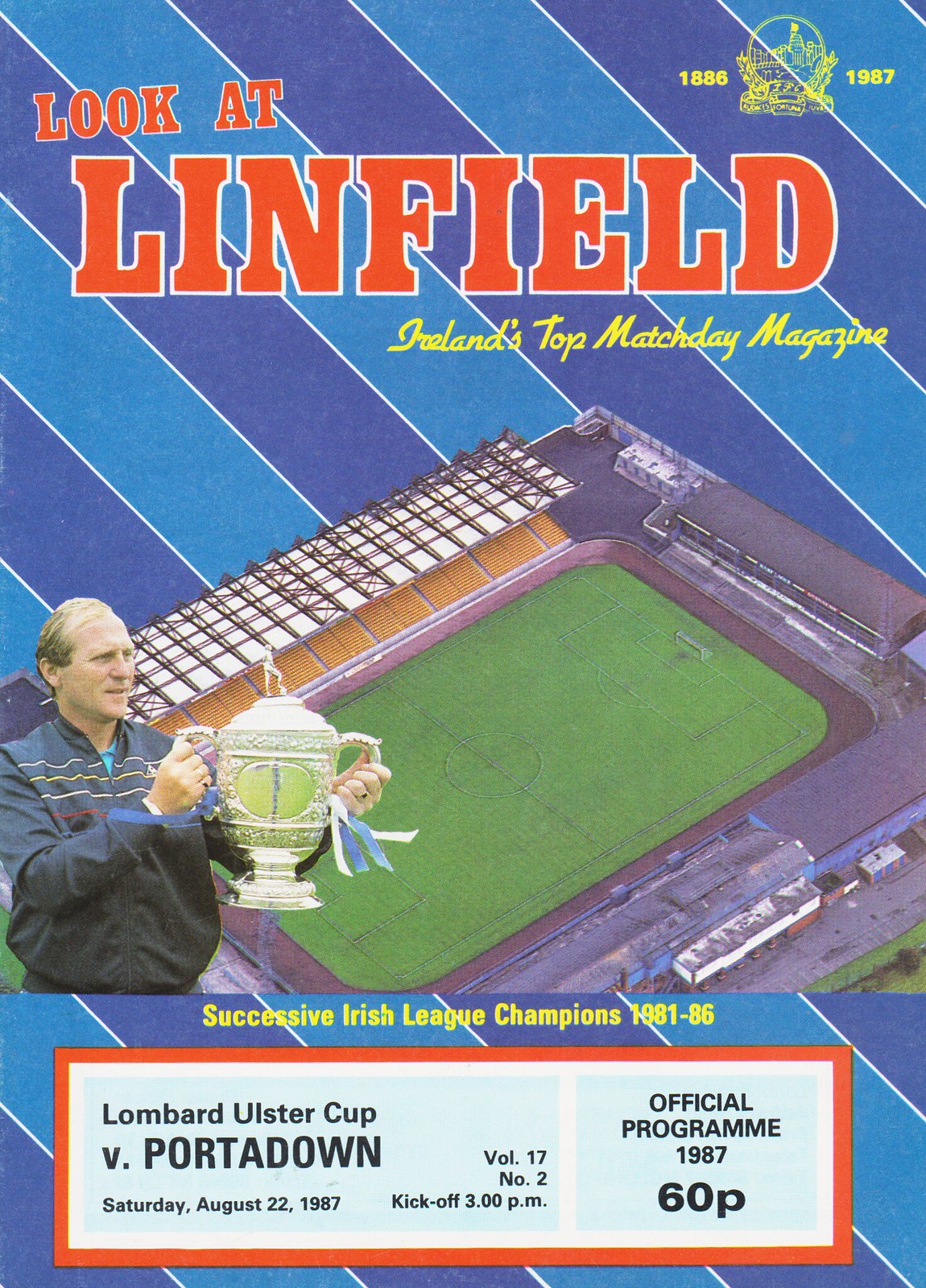The cover of the magazine, featuring imagery and text from Ireland's top match day magazine, "Look at Linfield," is designed with light and dark blue diagonal stripes. The title, emblazoned in bold red letters at the top, is followed by the subheading "Ireland's top match day magazine" in yellow. In the upper right corner, a logo indicates the years 1886 to 1987, marking the notable dates in the association’s history. The central focus of the cover is an aerial view of an empty soccer stadium, tilted at an angle, showcasing its white, gold, gray, and blue stands with a lush green field. Imposed over the stadium on the left is an image of a person in a dark blue jacket adorned with red, white, and yellow stripes, holding up a large gold trophy with blue and white streamers. Peach-skinned, the person is depicted triumphantly grasping the sides of the trophy. Below this, the text reads "Successive Irish League Champions 1981 to 86." Further down, in a white rectangle with a red border, it states "Lombard Ulster Cup vs Portadown, Saturday, August 22, 1987," followed by additional details: "Official Program, 1987, 60p" indicating the price, and "Volume 17, Number 2, Kickoff 3 p.m."